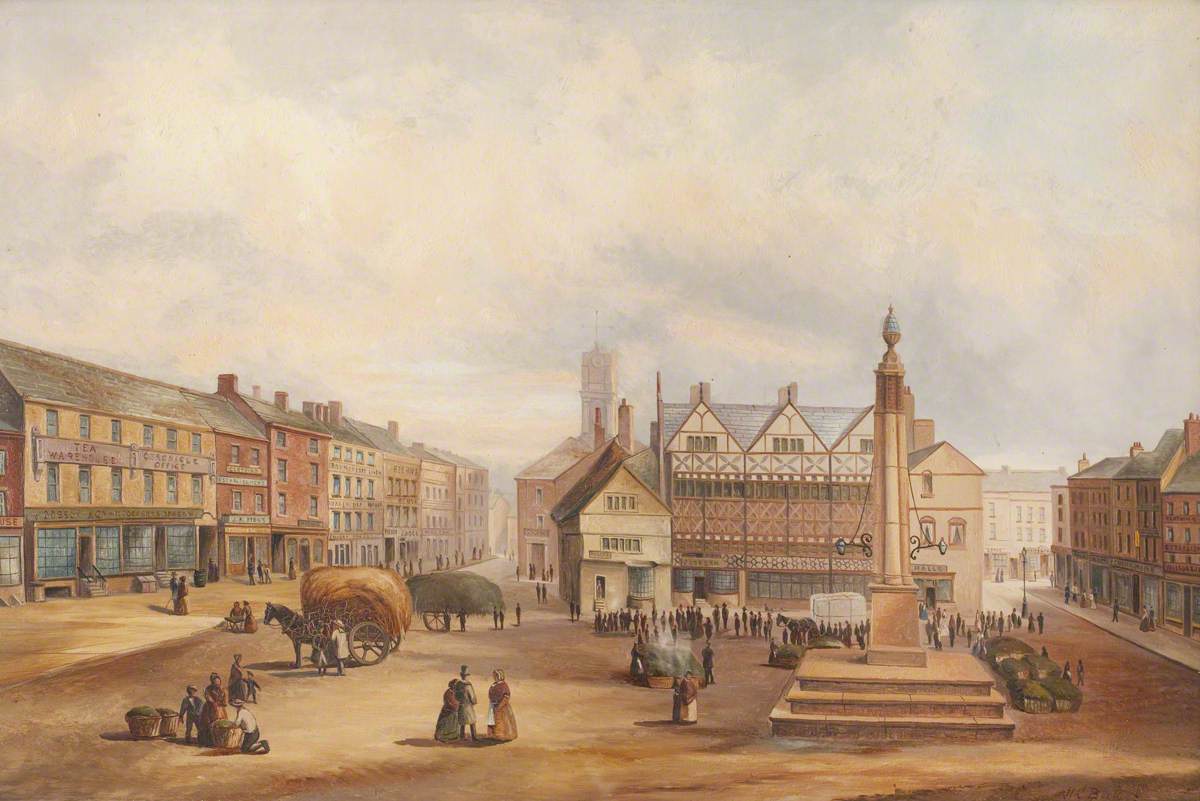The image captures an intricately detailed oil painting of an old-time city square, reflecting a bustling scene from the 1700s. Dominated by earthy tones of tan, brown, green, red, and white, the composition focuses on the town square situated in the bottom third of the painting. The square is animated with numerous people on foot and a few horse-drawn wagons – one notably loaded with loose hay. At the square's center stands a sculpture, surrounded by a variety of buildings, several of which rise to three or four stories high. To the left, right, and center, rows of houses frame the scene, while the background is capped by a partly cloudy sky. Among the notable buildings, a tea warehouse and what appears to be a post office are identifiable, lending a touch of historical authenticity to the bustling, urban atmosphere depicted in this beautifully rendered, old European or early American colonial city.